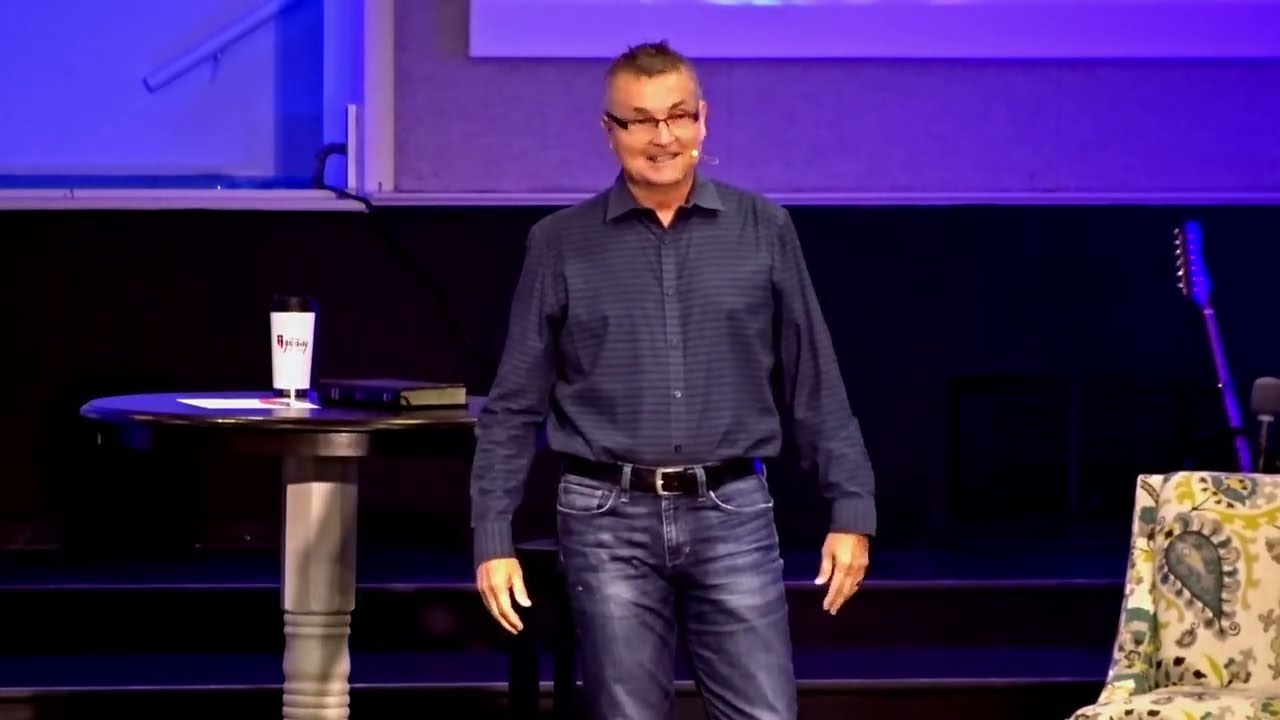In the center of the image is an older man standing on a multi-level stage, giving what appears to be a TED talk or a presentation. His attire includes a dark blue, long-sleeved button-down shirt with stripes, tucked into distressed blue jeans. He wears a black leather belt with a silver buckle, black-framed glasses, and has short brown hair. A small headset microphone is positioned near his mouth. The stage behind him is illuminated with blue and purple lighting, and the walls are black.

To the left of the man, there is a table with a white pillar base and a brown wooden top. On the table, there is a black book, potentially a Bible, and a white cup. On the right side of the man, there is a black chair with a floral pattern and the neck of a guitar, likely a bass guitar, is visible, indicating it is resting on the stage. There is also another microphone nearby. This indoor setting resembles that of an auditorium or performance venue, with the man seemingly addressing an audience.